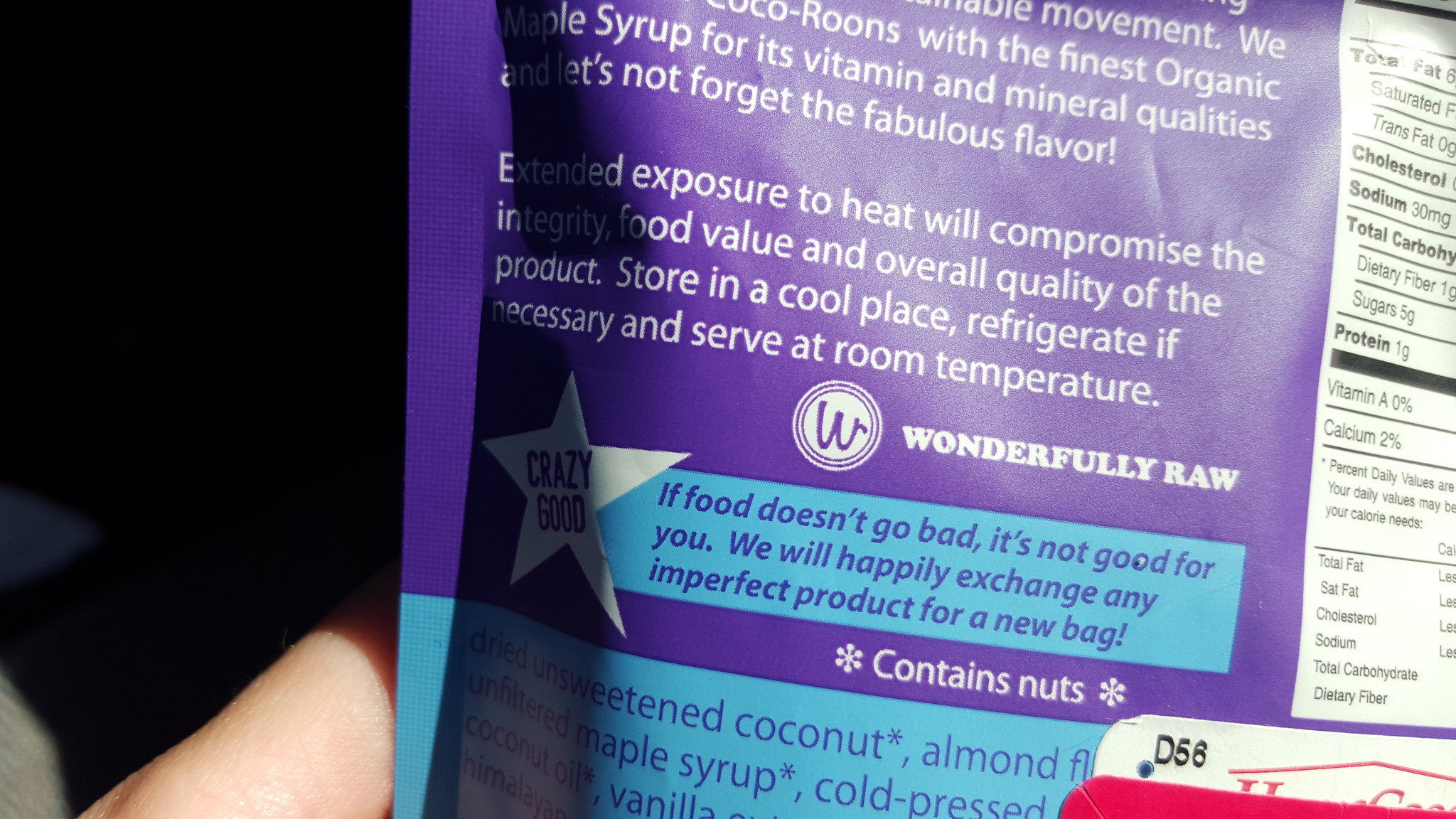This photograph features a close-up of a person’s hand holding the back of a food package, occupying about 60% of the frame. The skin on the visible parts of the fingers is Caucasian. The package has a predominantly purple main body with blue rectangular cutouts and assorted white and navy text. Notable details include a white star within a blue rectangle and a white circular emblem with a purple "W" in the center. The brand name "Wonderfully Raw" is prominently displayed in white font. Above this, smaller white text advises to store the product in a cool place, refrigerate if necessary, and serve at room temperature. Below, in navy font, the package states, "If food doesn't go bad, it's not good for you," accompanied by a promise to exchange any imperfect product for a new bag. 

The ingredients list includes items such as sweetened coconut, unfiltered maple syrup, and coconut oil, though not all ingredients are fully visible. Next to this list, a white rectangular nutrition label with black text provides partial nutritional information. The text also notes that the product contains nuts, marked with asterisks. The background behind the hand and package is entirely black, offering no additional detail. At the lower edge of the photo, partially obscured, are red and white cards encased or partially shown.